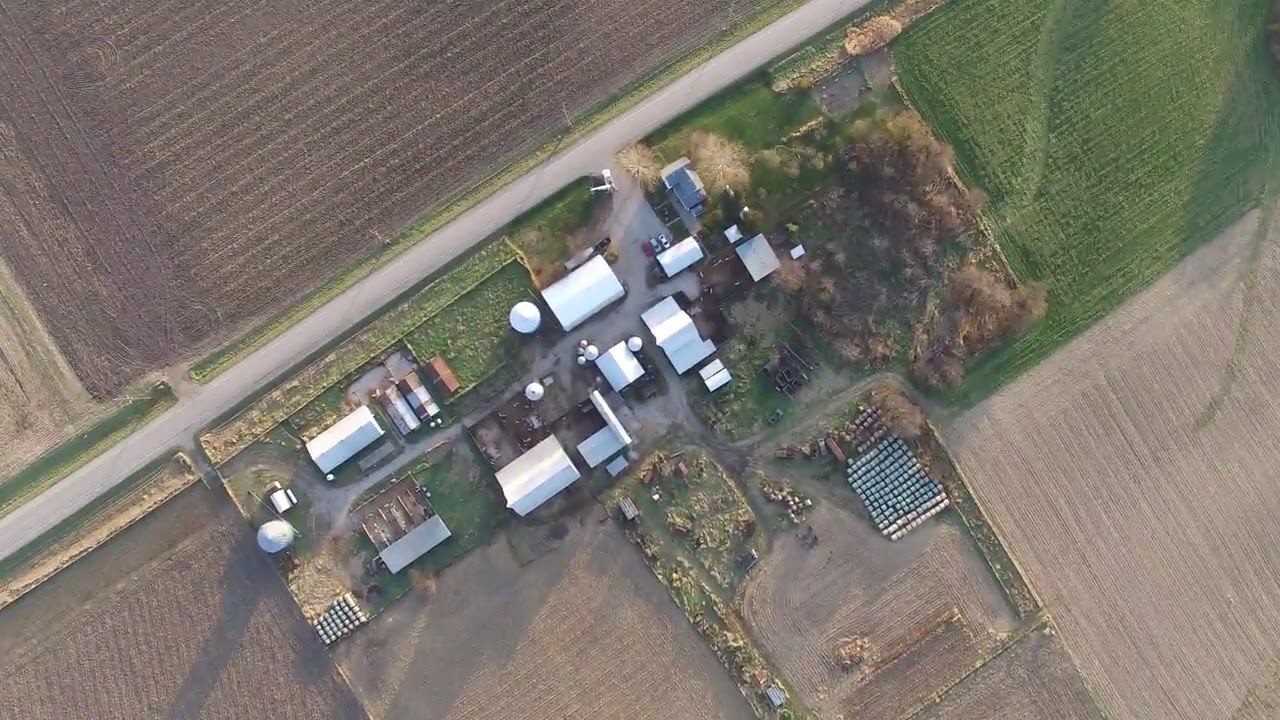An aerial image captures a sprawling farm scene showcasing various elements of agricultural and residential activity. On the right-hand side, there is a large expanse of tilled soil with visible planting rows, ready for sowing or perhaps already hosting crops like corn or beans. Above this area lies a stretch of meticulously maintained green grass. Dominating the middle of the frame, there is a cluster of white-roofed farm buildings including silos, barns, and equipment storage areas, with a few gray roofs and trailers interspersed. A dirt road cuts through this cluster, connecting the various structures and leading out to a main road that diagonally bisects the image from bottom left to top right.

To the bottom left of this central area, another set of buildings, possibly additional barns or outbuildings, stands with roofs varying from white to brown. Surrounding these structures are more fields, some appearing as light brown, freshly plowed soil fields, and others presenting as green expanses, possibly indicative of growing crops or pastures. Interspersed among these fields are patches of bushes and trees, sporting a mix of green and yellow foliage, adding natural variety to the landscape. The image lacks any textual signage, emphasizing the pure, outdoor essence of this active farm.